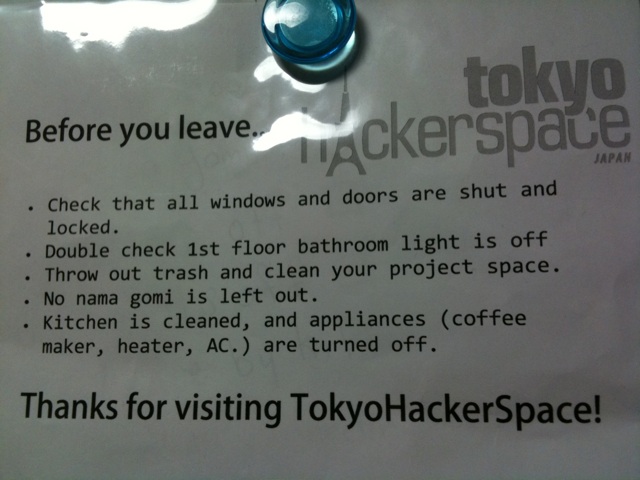The image depicts a laminated piece of white paper tacked up with a blue magnet. Despite the overall dull grayish tone of the paper, it shines slightly under some light. The text at the top reads "Before you leave" in large, black letters. Beneath that, on the right, in grayish text, it says "Tokyo Hacker Space" with the word "Hacker" stylized such that the 'A' resembles the Eiffel Tower. The word "Japan" is below, in much smaller text. The paper outlines five housekeeping rules in bullet points: 1) Check that all windows and doors are shut and locked, 2) Double check the first-floor bathroom light is off, 3) Throw out trash and clean your project space, 4) Ensure no namagomi (raw garbage) is left out, and 5) Make sure the kitchen is cleaned and appliances like the coffee maker, heater, and AC are turned off. The note concludes with "Thanks for visiting Tokyo Hacker Space!"